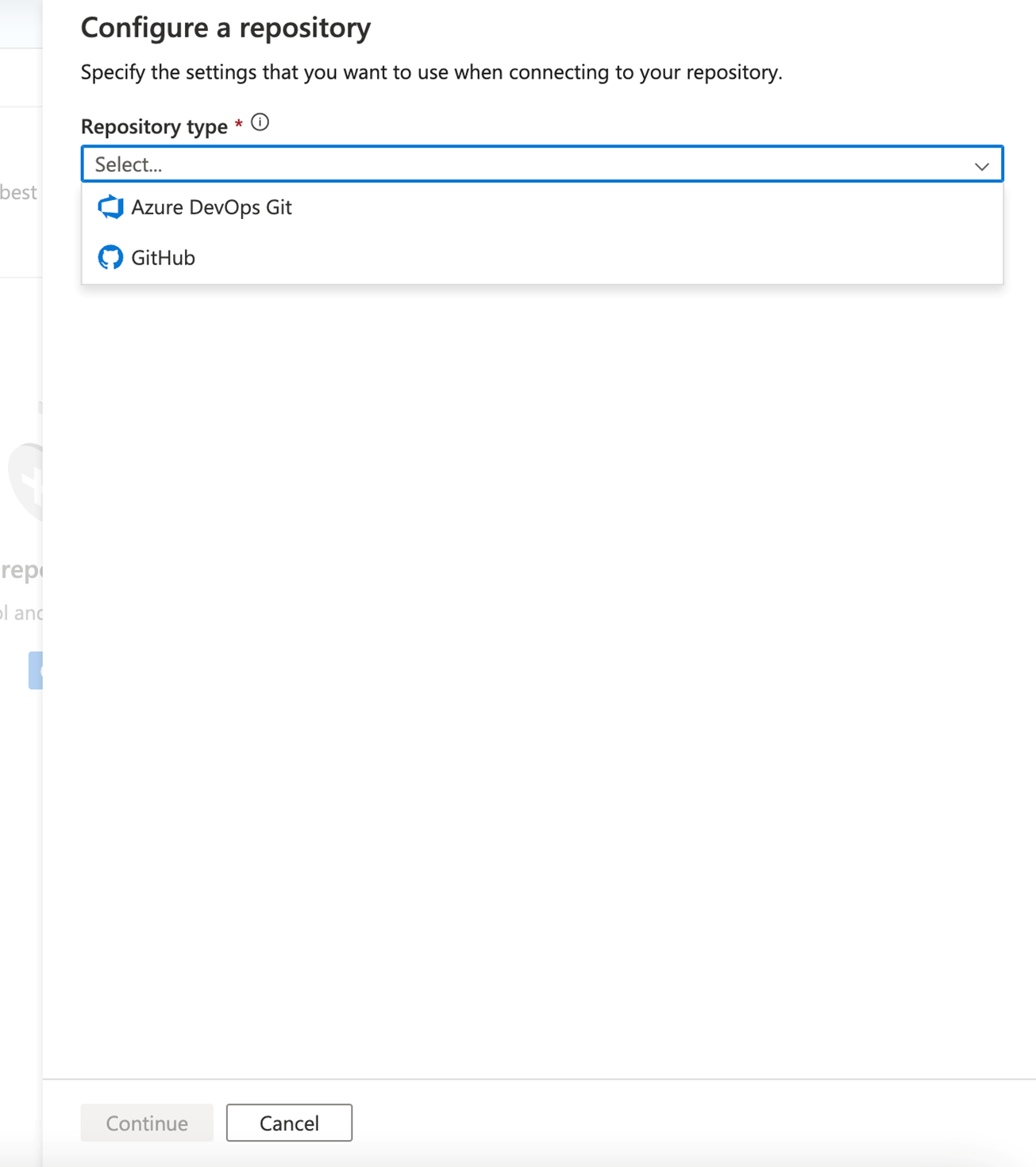The image features a user interface on a white background with a header reading "Configure a Repository." Below the header, the text prompts the user to "Specify the settings that you want to use when connecting to your repository."

Underneath this prompt, there's a label "Repository Type" accompanied by a small red asterisk, indicating a required field, and a gray circle with an "i" for additional information. 

Following this, a prominent blue dropdown box labeled "Select" with a downward arrow is visible. Within this dropdown, the options listed include "Azure DevOps GIT" and an option highlighted in blue titled "GitHub."

In the background, a partially visible box reveals text that includes the words "best" and "REP," along with a section of blue shading and a small blue mark towards the bottom. At the lower edge of the image, partial views of a "Continue" button and a "Cancel" button are discernible. Additionally, there's a small, indistinct mark located in the bottom right corner of the image.